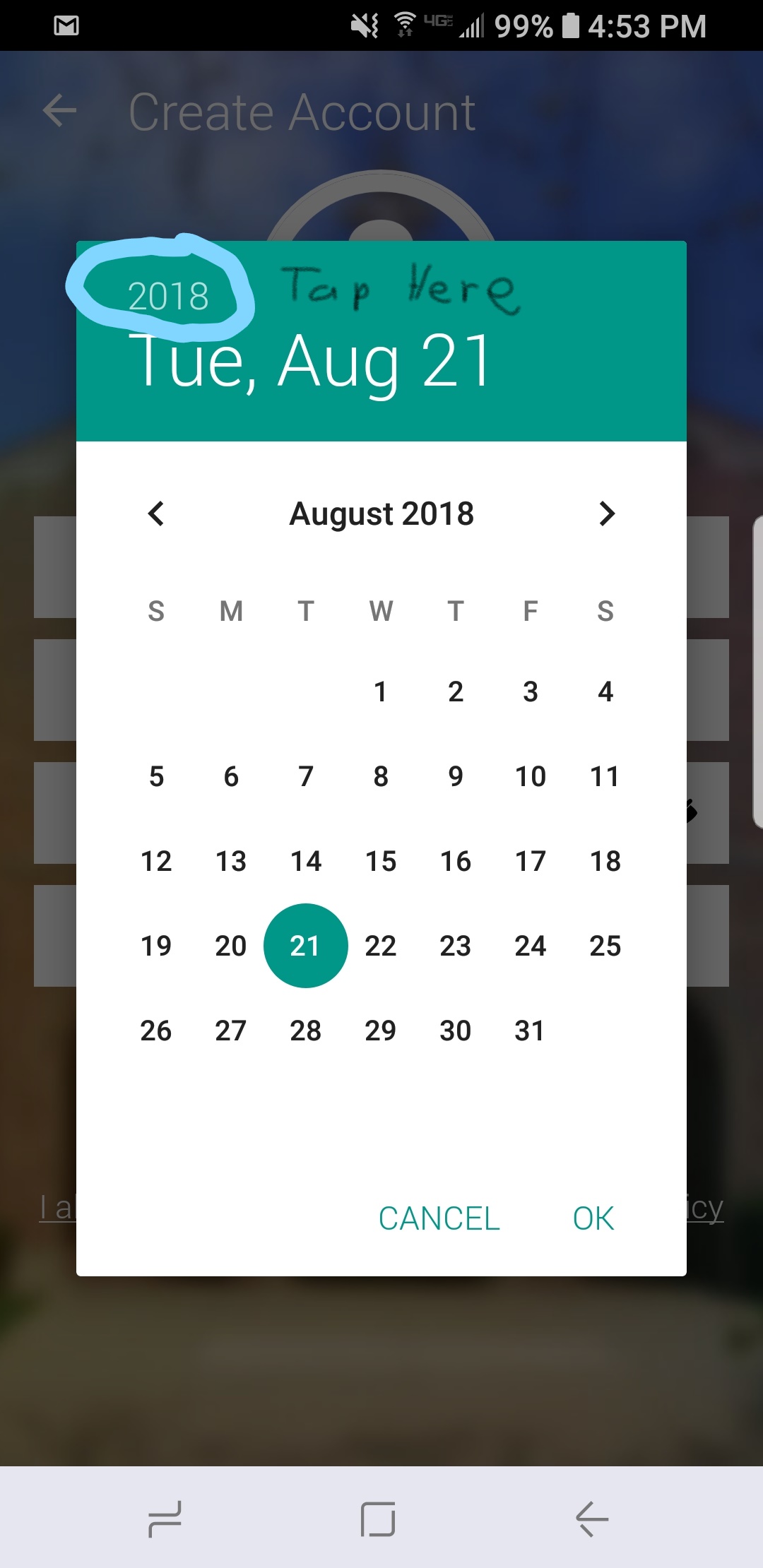The image depicts a screenshot from a digital calendar app on a smartphone, specifically showing the month of August 2018. In this screenshot, the date August 21st is prominently highlighted with a teal circle. Additionally, the year "2018" is circled in light blue ink, likely by a blue pen or marker. At the top of the calendar interface, the phrase "TAP here" is written in a somewhat child-like manner with unconventional capitalization: a capital "T", followed by lowercase "a p", then a capital "H", and finally lowercase "e r e". This text appears within a rectangular area containing the calendar display. 

Toward the bottom of the screen, there are teal-print buttons labeled "Cancel" and "OK", presenting options for user interaction. In the top section of the screenshot, a blue-colored area contains an arrow pointing left with the text "Create an account" or "Create account" adjacent to it. The time, displayed in the upper right-hand corner, shows 4:53 PM. The overall composition of the screenshot suggests that the user is either setting up or interacting with an event on the calendar.